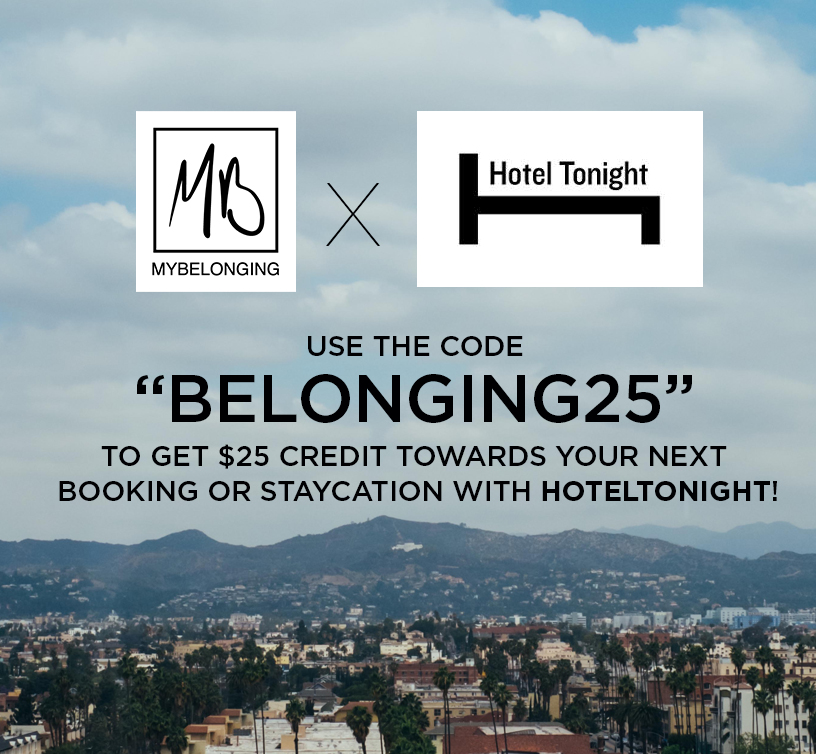Captivating aerial view of a serene Californian neighborhood captured in an advertisement. The image showcases a panoramic overlook of picturesque houses and buildings nestled among lush palm trees and undulating hills. A partially cloudy sky with hints of blue adds a dreamy, hazy ambiance, enhancing the quintessential Californian vibe.

Central to the image, a prominent white box presents the initials "MB" below which reads "My Belonging," pointing to a collaboration with another brand. Nearby, an 'X' subtly blends with the clouds, drawing attention to a second white box featuring a sideways silhouette of a bed. Above this bed, text declares “Hotel Tonight.”

Emblazoned on the clouds with black writing, the promotional offer stands out: “Use the code ‘BELONGINGS25’ to get $25 credit towards your next booking or staycation with Hotel Tonight!” This compelling message encourages viewers to take advantage of this exclusive offer, emphasizing the partnership between "My Belonging" and "Hotel Tonight" and urging them to explore a seamless, enjoyable staycation experience.